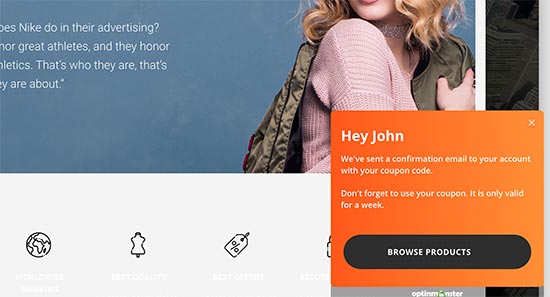This image depicts a partially visible webpage featuring a fragmented headline that reads "Nike," followed by an incomplete phrase and a question mark, which repeats across four lines. The background of the webpage is a light blue hue. On the right side of the image, there is a cut-off photo of a woman whose face is mostly obscured, but you can see her from the bottom lip downwards. She has blonde hair that falls on both sides of her face. The woman is Caucasian, wearing a pink sweater and a greenish jacket while crossing her arms. She also dons what appears to be a choker-like necklace.

Overlaying the image in the top right corner is an orange square box with the text "Hey, John" in it, followed by two short paragraphs underneath. There is also an oval-shaped, black button labeled "Browse the products" situated below the text.